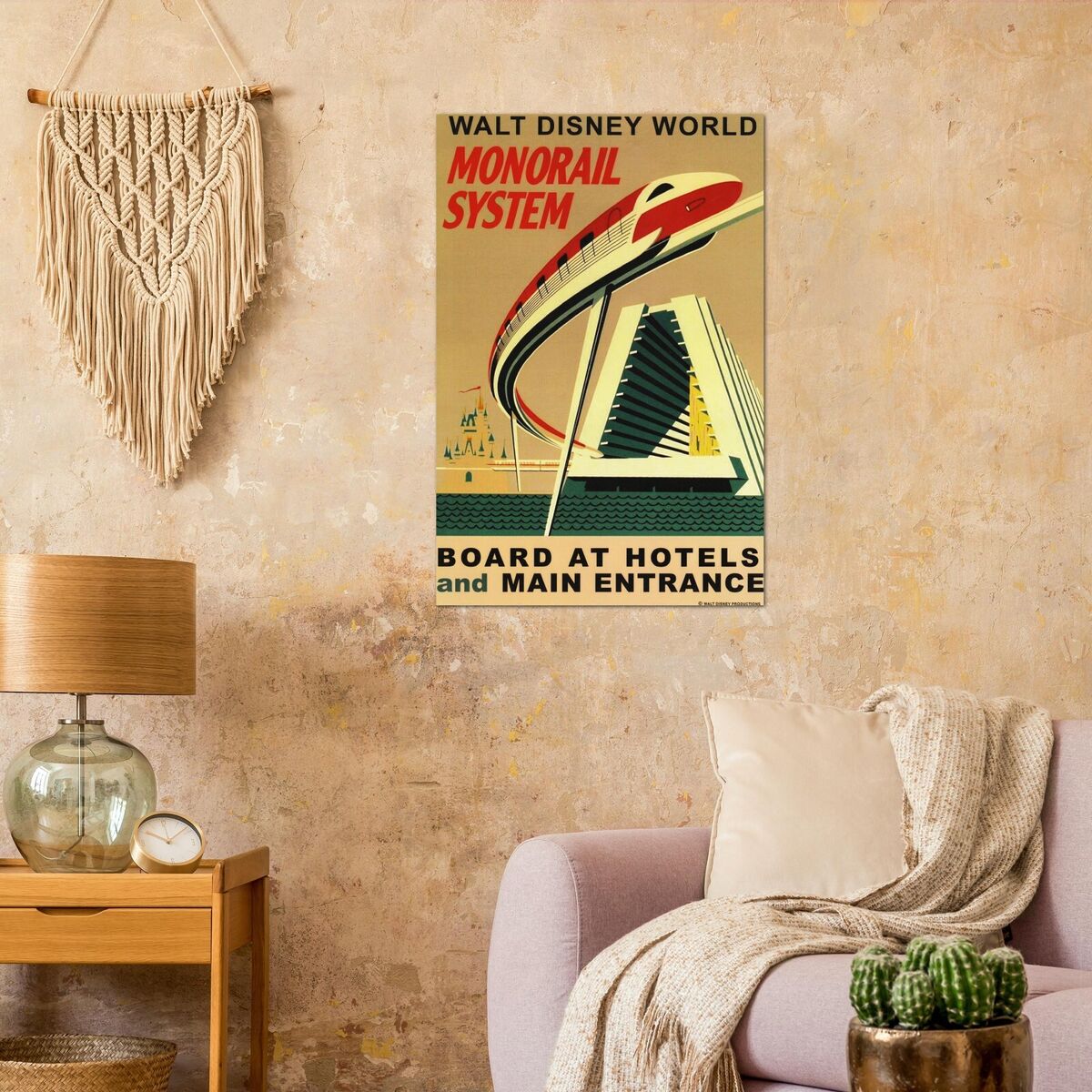The image resembles a meticulously arranged advertisement scene, capturing a cozy living room corner with a perfect, almost idyllic setup. The central focus of the space is a lilac-colored couch adorned with a tan pillow and a draped tan throw. A golden pot holds a cactus, positioned on an unseen table in the lower right corner. Adjacent to the couch in the lower left, a small, brown side table with a basket beneath it hosts a glass lamp with a wooden shade and a small clock. Hanging prominently on the wall above the table is a beige macrame design. The wall itself is a worn, multi-toned canvas featuring hints of tan, white, dark brown, and orangey yellow, contributing to the room's artistic ambiance. Centrally displayed on the wall is a poster reading "Walt Disney World Monorail System, board at hotels, and the main entrance," depicting the monorail exiting the Contemporary Resort. This vintage-style poster emphasizes the room's perfect blend of comfort and nostalgia, making it reminiscent of a Disney World advertisement.